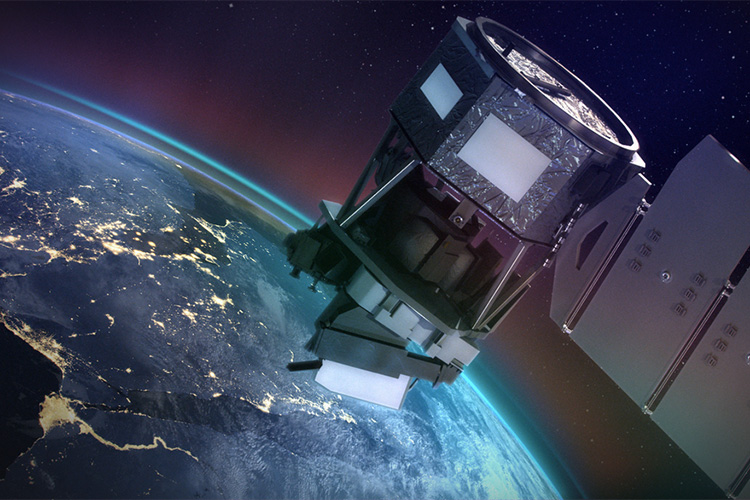This rectangular, landscape-oriented image, approximately 6 inches wide by 4 inches high, depicts a satellite orbiting Earth. The photograph captures the satellite front and center, facing towards the planet. The satellite is predominantly black with multiple components, including metal bars and an electronic assembly; its bottom part reflects blue light from Earth. The satellite has a roundish structure covered in silver, reflective material, and a large flat panel extending to the right.

Positioned in the lower left portion of the image, the planet Earth occupies roughly a quarter of the frame, displaying its spherical curvature. The planet's atmosphere is a thin, glowing band of bright blue encircling it. Earth's surface features a variety of colors including blue, gray, and light brown, with distinctively white lines visible.

The background of the image is the expanse of outer space, beginning around Earth with a light pinkish-purple hue that transitions to deeper purples and blues. Scattered throughout the sky are numerous white dots representing distant stars. The overall scene combines the detailed foreground of the satellite and the expansive, colorful depiction of Earth and space.